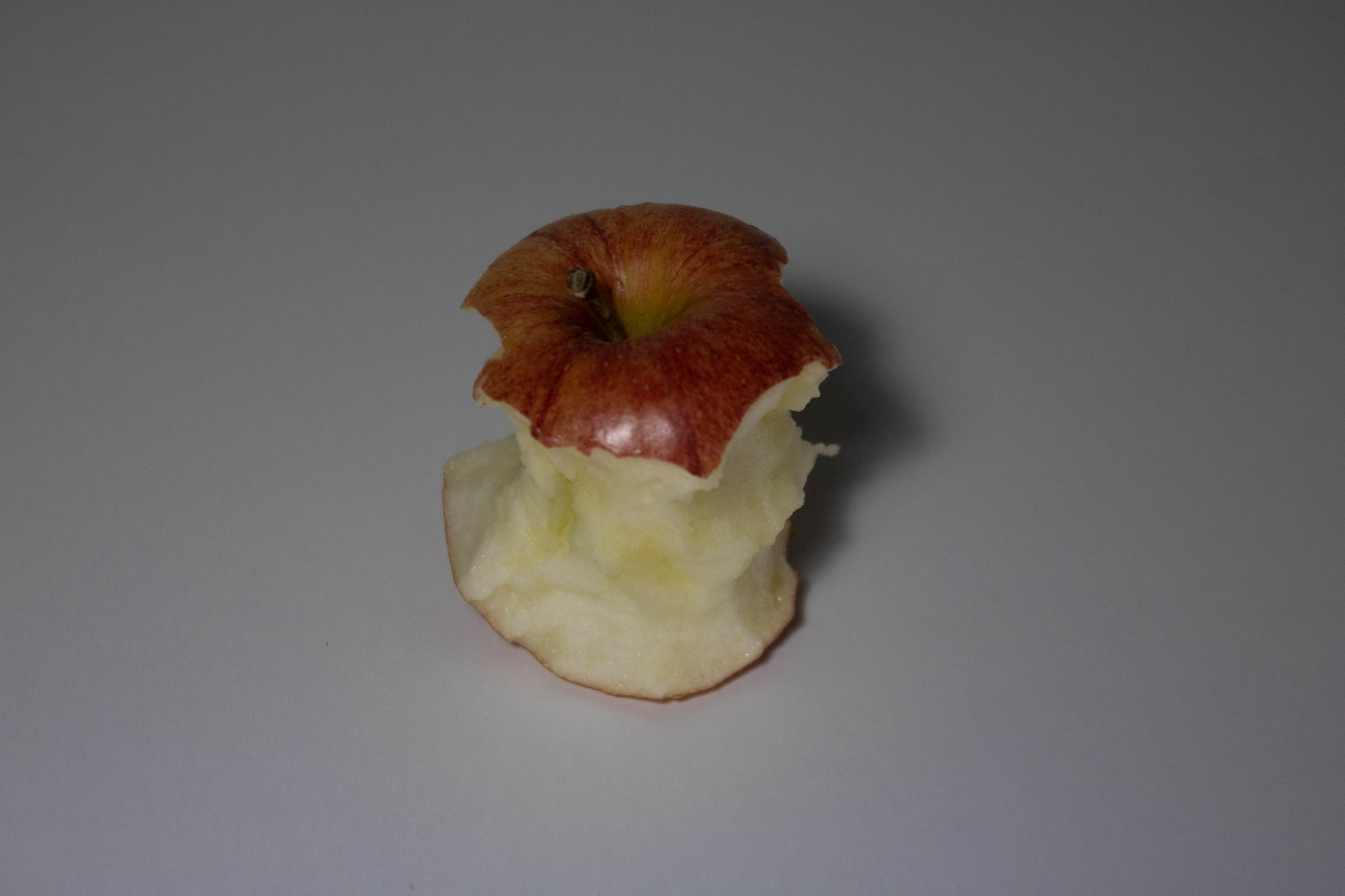This is a professional, color photograph capturing a nearly consumed red apple, centered perfectly within the horizontal, rectangular frame. Approximately 80% of the apple has been eaten, exposing its core and a whitish flesh that shows signs of oxidation with patches of yellowish-brown discoloration. The brown stem juts out from the top, a stark contrast against the lush, red peel encasing the remaining sections of the fruit. Subtle details, such as a small shadow on the apple's upper right-hand corner and bits of moisture forming around the bottom right-hand area, amplify its realism. Additionally, a piece of the apple's peel is still attached at the bottom, grounding the apple as it sits upright. The overall composition and lighting suggest a meticulous, professional approach to photography, enhancing the visual appeal of this simple, yet evocative subject.